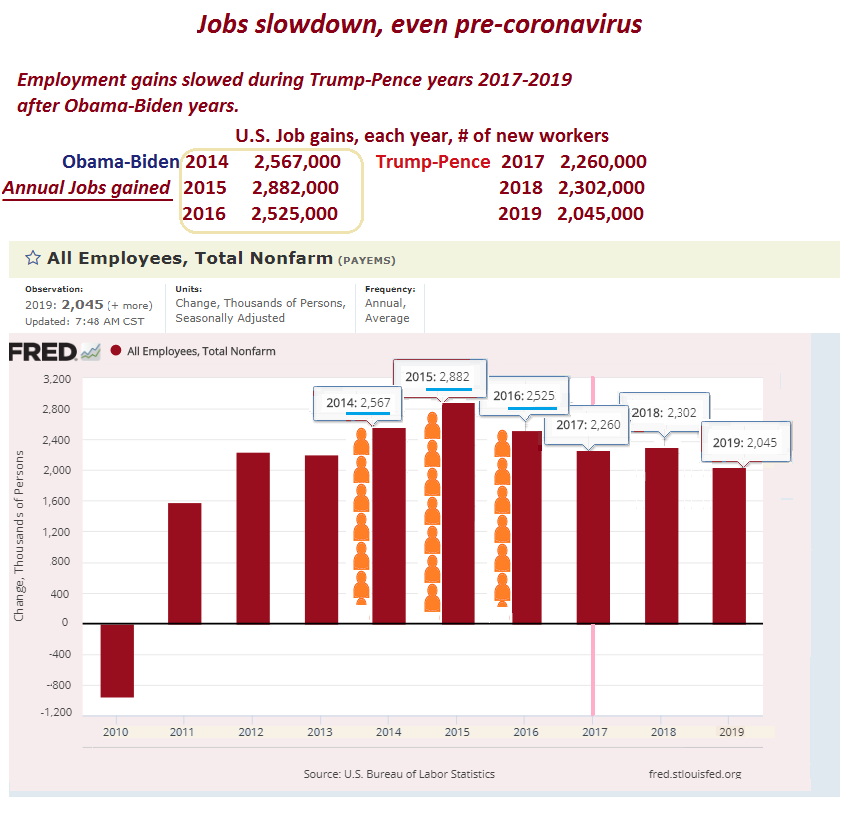The image depicts a bar graph with the title "Jobs Slow Down, Even Pre-Coronavirus" prominently displayed at the top. Below this, it states, "Employment gains slowed during Trump-Pence years (2017-2019) after Obama-Biden years." The graph is labeled "U.S. Job Gains Each Year: Number of New Workers" and includes detailed numeric data comparing job gains between the two administrations. For Obama-Biden, the job gains are listed as follows: 2014 - 2,567,000; 2015 - 2,882,000; 2016 - 2,525,000. For Trump-Pence, the numbers are: 2017 - 2,260,000; 2018 - 2,302,000; 2019 - 2,045,000. 

The graph itself features vertical bars in maroon red with corresponding values placed on top. On the left axis, the numbers range from 3,200 down to negative 1,200, with the label "Change in Thousands of Persons" running vertically. The horizontal axis spans from 2010 to 2019. At the very bottom, it cites "Source: U.S. Bureau of Labor Statistics," with additional attribution to "Fred St. Louis Fed.org" on the right side. The section in maroon red labeled "All Employees, Total Non-Farm" captures broader employment trends depicted on the graph.